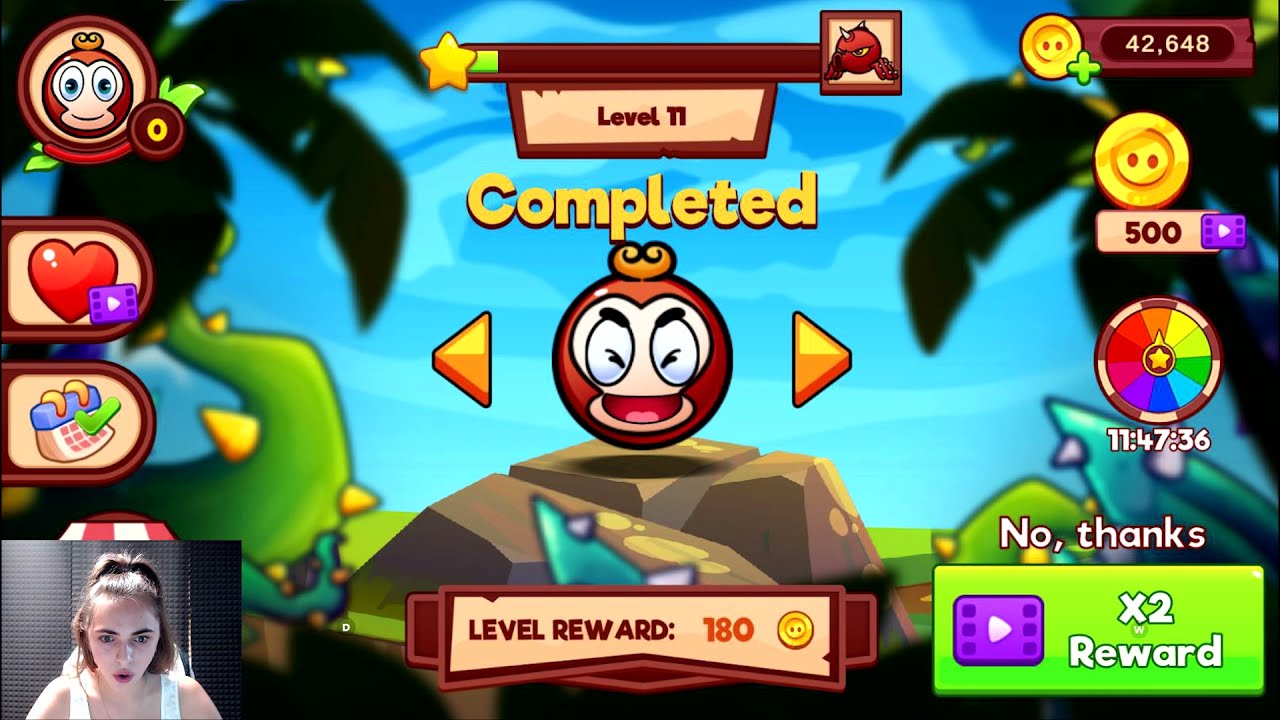An image captures a cheerful, cartoony app game being streamed by a white woman wearing a white tank top with her hair tied back, appearing in a small video window at the bottom left corner. Her expression is one of excitement and surprise, her mouth slightly open as if she's speaking. The game's main screen, set against a light blue background adorned with palm trees in the corners, displays vibrant action. At the center of the screen, yellow text reads "Level 11 Completed" above a smiling, monkey-like character with large eyes. Flanking the character are yellow arrows. In the top left corner, icons including a heart and a calendar are visible, while the right side features a colorful spinner icon and a money symbol. The bottom of the screen includes a section with "Level Reward 180" next to a gold coin icon in the center, and a "No Thanks" button coupled with a video icon offering "x2 reward" in the lower right corner.